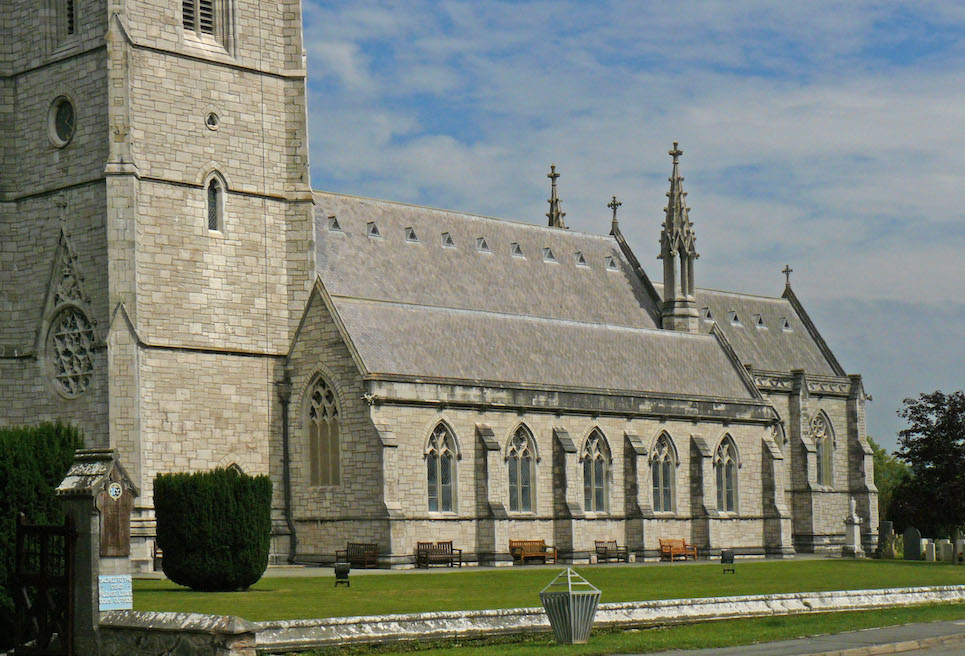This image depicts a large, historic stone church, unmistakably identifiable by the prominent crosses atop its multiple spires. The building is constructed from varied gray stones, each unique in size and shape, adding a rustic charm. Its tall, triangular gray roofs and pointed gothic architecture evoke a sense of grandeur and antiquity. Distinct features include the domed windows on the main structure and a smaller rectangular building attached to the right, enhancing the layered architectural complexity. The left side boasts a towering spire, much taller than the rest of the edifice, contributing to the church’s commanding presence.

The scene includes a vibrant green lawn in the foreground, interspersed with wooden benches for visitors. A small graveyard with tombstones is visible in the lower right, bordered by shrubs and partially enclosed by a stone wall and pillar, hinting at the church's age and the community it serves. The serene blue sky dotted with white clouds complements the peaceful ambiance. This detailed portrayal, capturing elements of both old-world gothic design and a well-maintained surrounding landscape, suggests the image might be artistically rendered rather than a photograph, given its vibrant yet slightly surreal qualities.